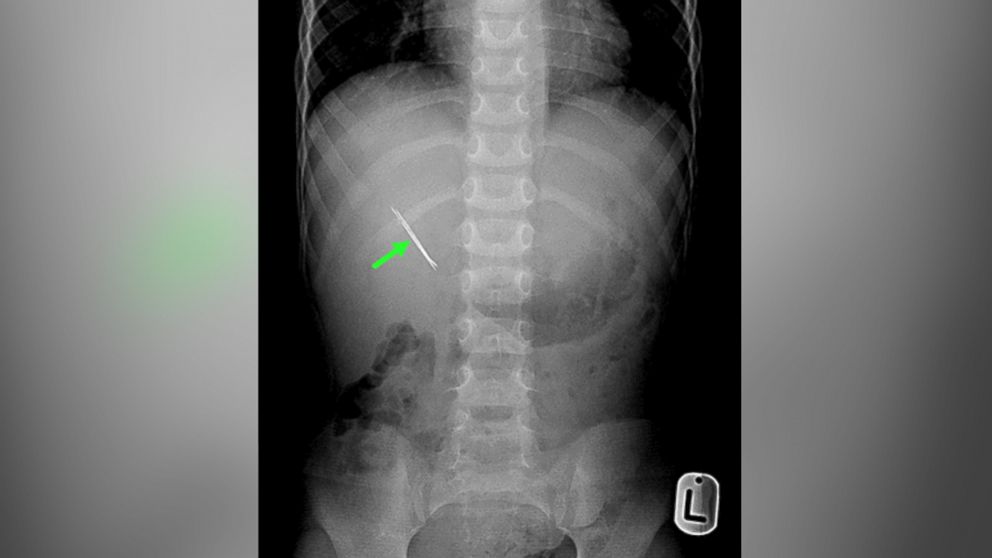This is an x-ray image of a torso, depicting the spine, ribs, and pelvis in luminous white against a pitch-black background. The spine stands out prominently, glowing white along the vertical center. In the bottom right corner, there is a marker resembling a dog tag, with the letter "L" printed in black. To the right side of the image, near the lung area, there's a computerized green arrow pointing at a solid white object that appears to be lodged at a 40-degree angle within the ribcage or lung. This large slit-like object contrasts starkly against the typical cloudy gray and white hues of the x-ray. Given the slender anatomy and additional context, the image might be of an animal—possibly a dog—taken either at a veterinary clinic or a medical office.